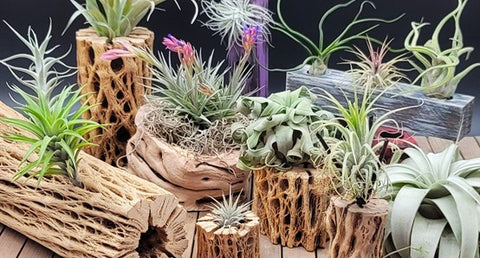The image showcases a detailed, intricate display of various succulents and desert plants, many of which are emerging from stylized driftwood and decaying wooden logs. The plants feature wiry, crazily shaped leaves and exhibit a range of colors, primarily pale green, light gray, and vibrant shades. Most of the plants are placed on wood slats against a plain, dark blue background. Notably, a cylindrical piece of wood on the left side has a green plant with thin, multi-directional leaves, which are paler at the top and more vibrant at the bottom. Among the diversity, there are plants with tentacle-like appendages and some with purple or lavender blooms, alongside a narrow-leaved bromeliad coming from the center of dried logs. The foreground features a fern-like, light gray bromeliad with an intricate, interwoven appearance. This scene could easily be part of a terrarium display, combining elements of desert and underwater plant aesthetics.